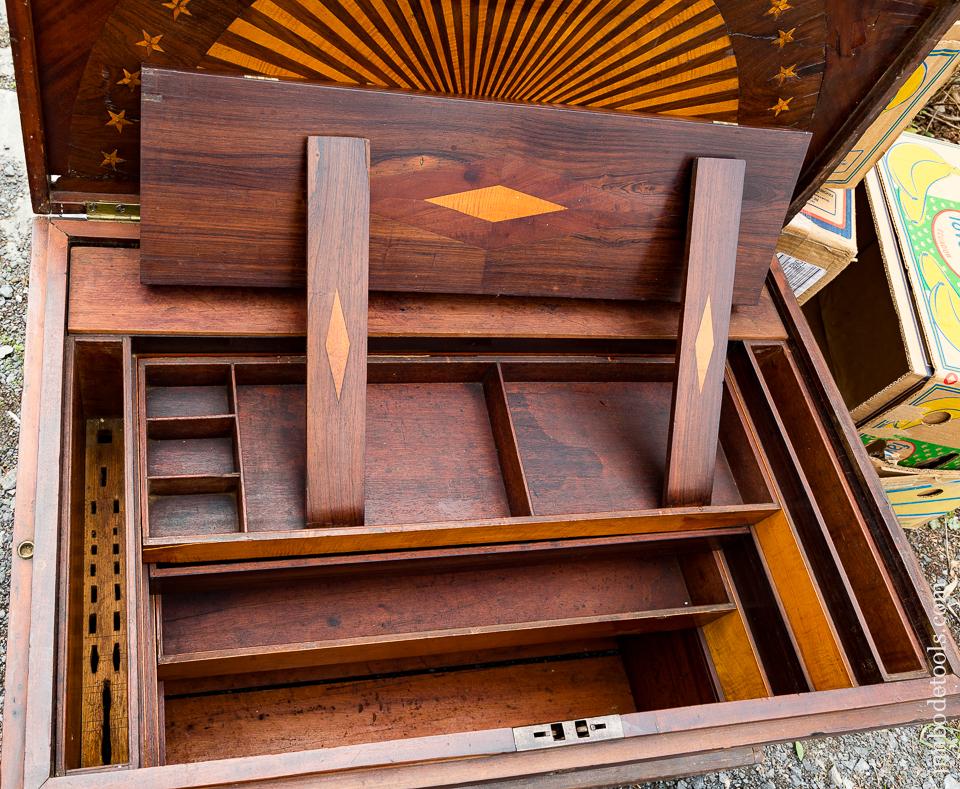This image depicts an old-fashioned wooden chest, likely photographed outdoors in a gravel-strewn area next to a green and yellow banana box. The chest is made entirely of wood, featuring a mix of different-colored woods such as blonde, light tan, and dark woods, which accentuate its vintage design. The chest is open, viewed from a top-down angle, showcasing multiple thin, removable drawers or trays inside. Two flat pieces of wood, adorned with diamond patterns and lighter hues, are propping up the lid, suggesting that the chest might be undergoing some repairs. The inside of the lid also displays an elaborate design with gold star patterns arranged in a half-circle and what resembles a fan-shaped motif with ray-like streaks extending outward, adding a touch of elegance to this rustic piece. Overall, this gives the impression of a meticulously crafted and storied item, blending utility with ornamental artistry.